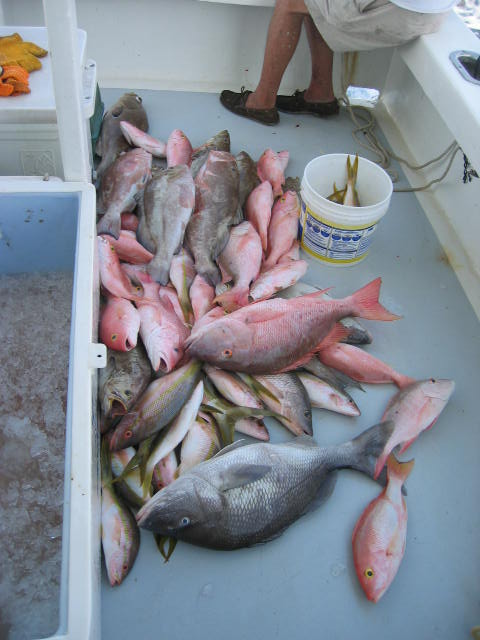The image depicts the chaotic scene of a fishing boat's deck, strewn with freshly caught fish of various colors, predominantly pink and gray. These fish lay haphazardly across the floor, some with mouths ajar, creating a vivid tableau against the boat's grayish-blue bottom and white sides. In the corner of the boat, a person sits on the side rail, identifiable by their light beige shorts and brown shoes, though their upper body is partially cropped out of the frame. Nearby, a white cooler filled with ice stained reddish with blood hints at the recentness of the catch, while a bright pair of yellow and orange gloves rest atop another cooler. A sturdy rope, likely linked to an anchor, snakes its way across the deck, and a silver fishing pole holder is mounted on the boat's side, further emphasizing the vessel's purpose. The overall scene captures the essence of a bustling fishing expedition, rich in detail and color.